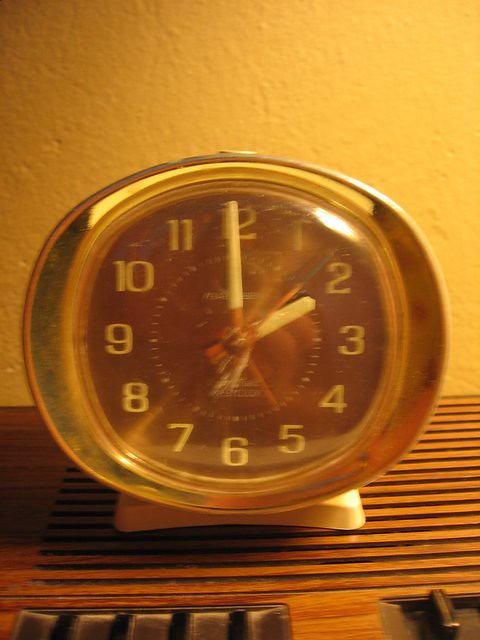The image features an old-style alarm clock, reminiscent of the 1960s or 70s, with a somewhat oblong shape. The clock rests on top of an old-fashioned sound system or TV, which is characterized by wood grain texture with divots and knobs, as well as black buttons on the right and a small lever in the corner. Bathed in a warm, orange glow from a nearby light bulb, the clock has a silver rim encircling a dusty glass front. The clock face, which is black with white numbers from 1 to 12, features distinct white hands with red bases, and a unique rainbow-colored second hand transitioning from red to yellow to green. The whole scene is set against a subtly textured, plaster wall that appears yellow under the lighting. The time displayed is 1:59, with the second hand pointing at the five.